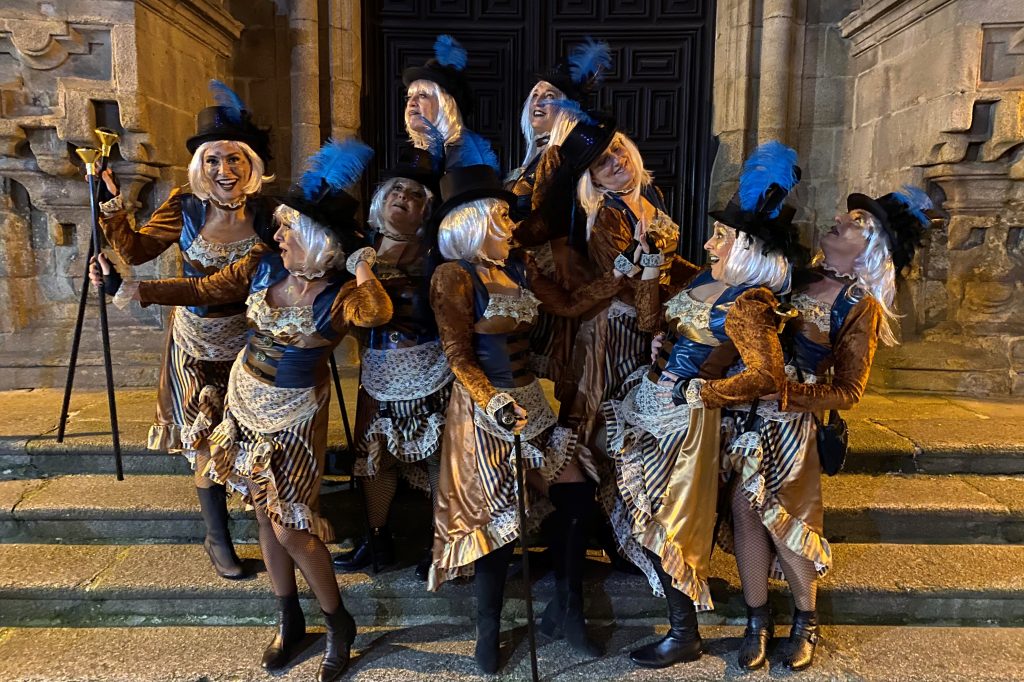The image displays a group of nine women standing on three wide steps in front of a stone building. They are all dressed identically in early 1920s-style gold and black dresses, complemented by black ankle boots. Each woman sports a blonde wig topped with a black hat adorned with a blue feather. Some of them are holding canes, and they strike various cheerful poses suggesting camaraderie, possibly indicating they are part of a theater or dance troupe. The photo appears to have been taken at night, adding a dramatic touch to the scene, which bears the hint of being either a painting or a retouched photograph.